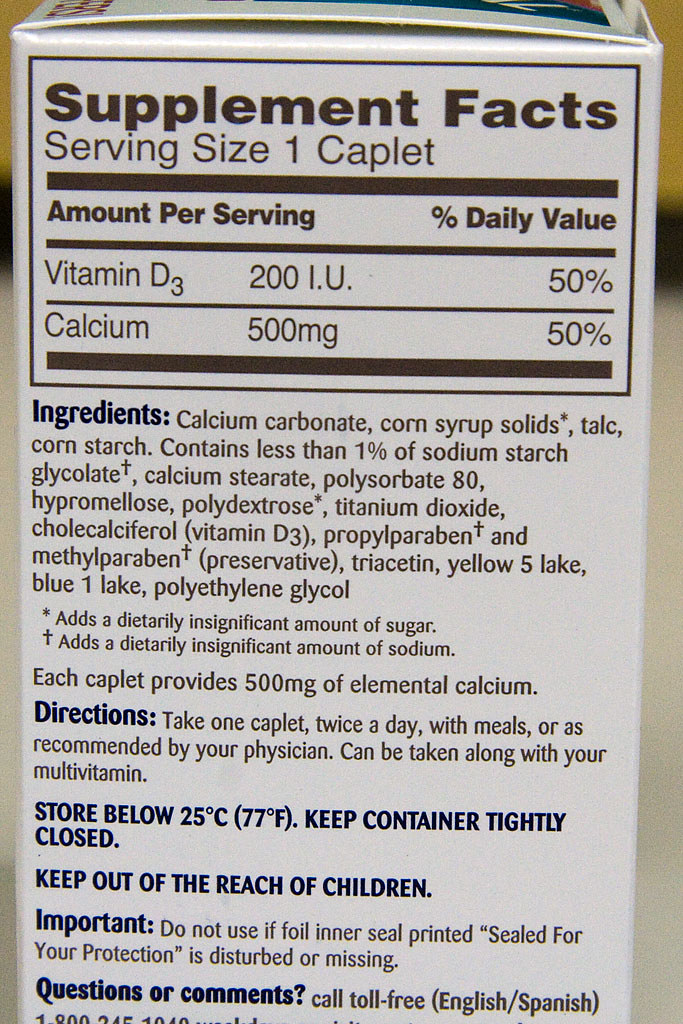Photograph of the Supplement Facts on the Back of a Cardboard Box

The image features the back of a cardboard box prominently displaying the supplement information. The "Supplement Facts" are labeled in bold, black letters within a black-outlined rectangle. The serving size is listed as one caplet. It specifies the intake amounts for Vitamin D3 and Calcium per caplet.

Beneath the supplement facts, a section titled "Ingredients" is highlighted in bold blue letters, followed by a detailed list of the ingredients in smaller, non-bold black font.

Below the ingredients section, another header in bold blue letters reads "Directions." In smaller, non-bold black text, the directions instruct to take one caplet twice daily with meals or as advised by a physician, along with additional usage recommendations.

At the bottom, in large, bold letters, it advises to "Store below 25 degrees Celsius" and to "keep container closed tightly." There are also some other directions and warnings included in the lower portion of the box.